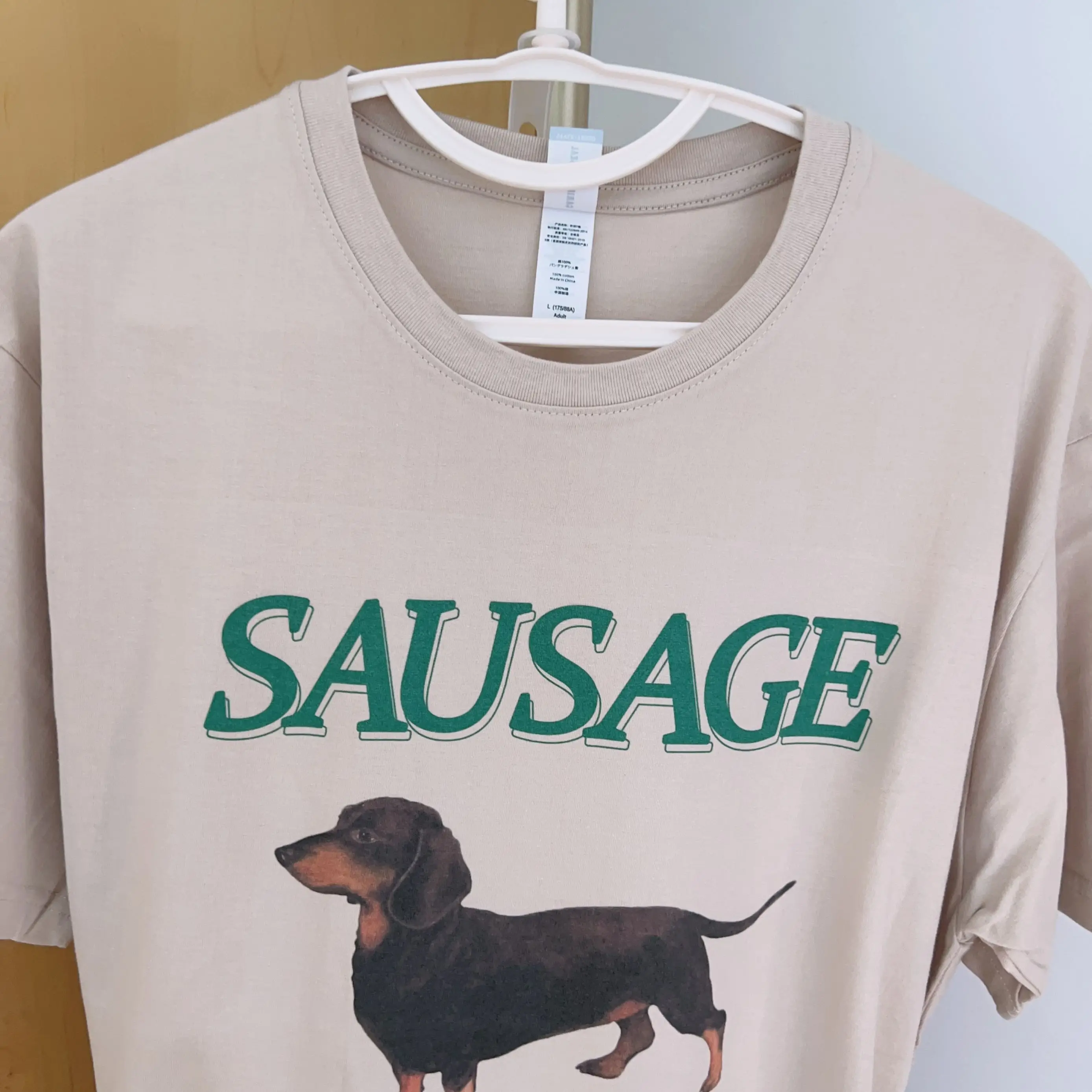A short-sleeved, light grey graphic t-shirt is hanging from a white, curved hanger, which itself is hung on a white, light-colored wooden door, set against a white painted wall. The shirt features a vibrant green print of the word "sausage" across the chest, accompanied by an illustration of a dachshund—a wiener dog with short, stubby legs that are light brown, a long black body, a pointed black tail, and floppy black ears. The dog's snout and upper neck are also light brown, contrasting with its black head and body. Adding a touch of novelty, the shirt has a white tag at the collar, partially flipped up, likely detailing the washing instructions. The overall impression is one of good-natured humor, making the shirt a fun, casual piece.